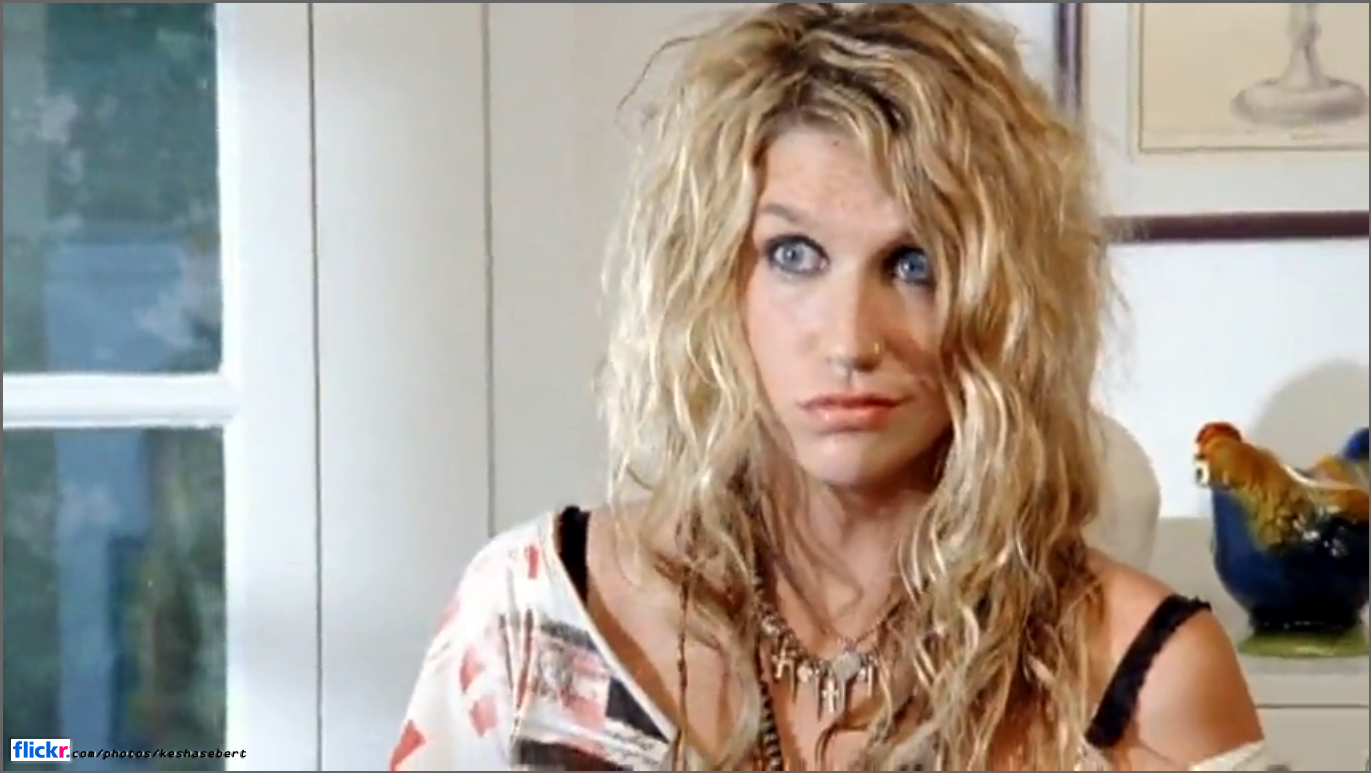This photograph captures Kesha Siebert from the chest up, her long, messy blonde hair cascading over her shoulders in wavy, curly strands. She wears a black garment with visible straps that suggest a tank top or bra, partially obscured by a white shirt adorned with a graphic design in black, red, and white. Around her neck hangs a necklace adorned with numerous charms, including crosses and circles. Kesha's expression is one of perplexity, with a questioning gaze directed past the camera. The background features a table with a ceramic rooster, a white wall with a framed pencil sketch in a gray frame, and the paned glass of a door or window. The bottom left corner of the image is marked with "Flickr, COA/photos/Kesha Siebert."